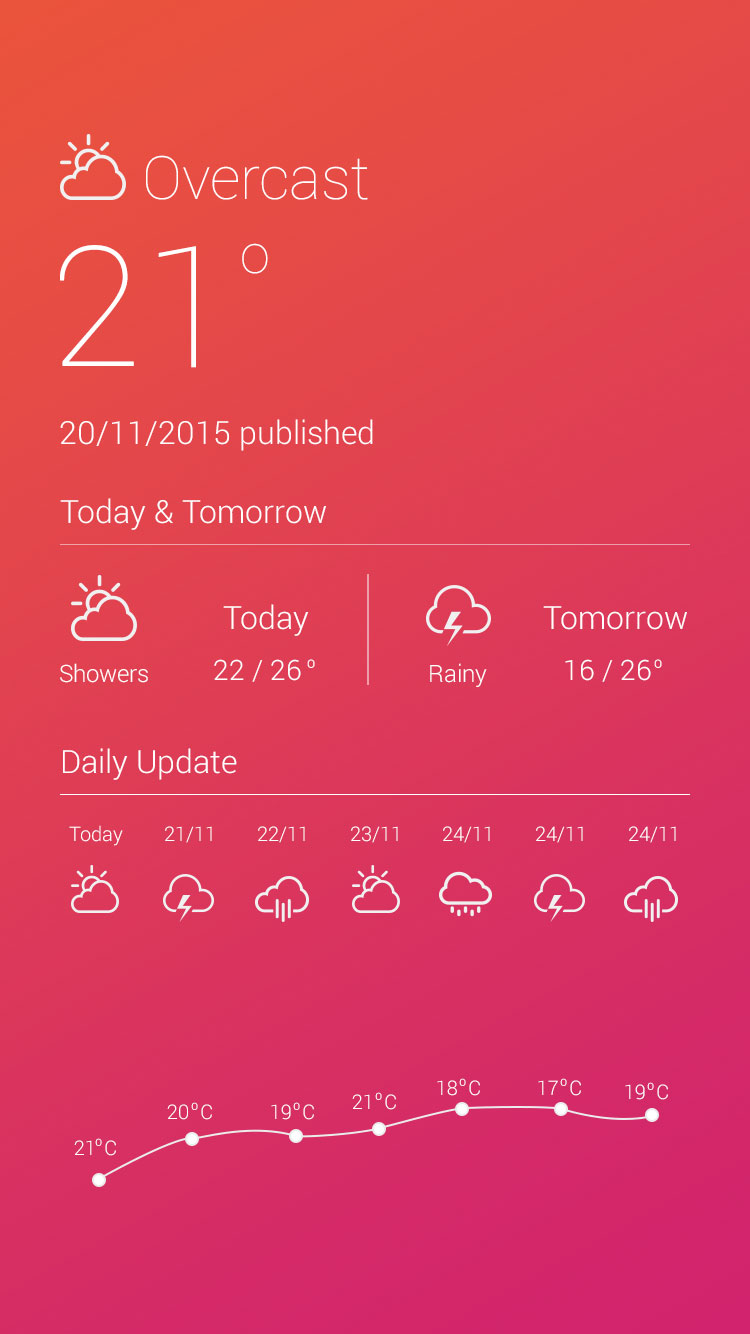This image is a cropped screenshot of a weather app on a mobile phone. The user interface elements of the phone itself (top and bottom bars) are not visible in this screenshot. 

At the top, the app displays the weather condition as "Overcast" with a small graphic showing a sun partially obscured by a cloud. Immediately below this, the current temperature is prominently displayed as "21°C". 

In smaller text beneath the temperature, the date of publication is noted as "20/11/2015". Following that, there's a section labeled "Today and Tomorrow," which provides a brief forecast for the day and the next.

On the left side, the forecast for today shows temperatures ranging between 22°C and 26°C, with an indication of "showers" accompanied by a cloudy sun symbol. To the right, the forecast for tomorrow is presented with a thundercloud icon, indicating "rainy" weather with temperatures from 16°C to 26°C.

Below this, there's a section titled "Daily Update" with a sequence of dates listed (21/11, 22/11, 23/11, 24/11, 24/11, and 24/11). Beneath these dates, a dotted line graph visually connects several data points, representing the temperature forecast over the specified days.

The background of the screenshot transitions from a warm red at the top to a cooler purple at the bottom, with intermediate shades of peach. All text and graphical elements within the app are rendered in white against this gradient backdrop, ensuring clarity and contrast.